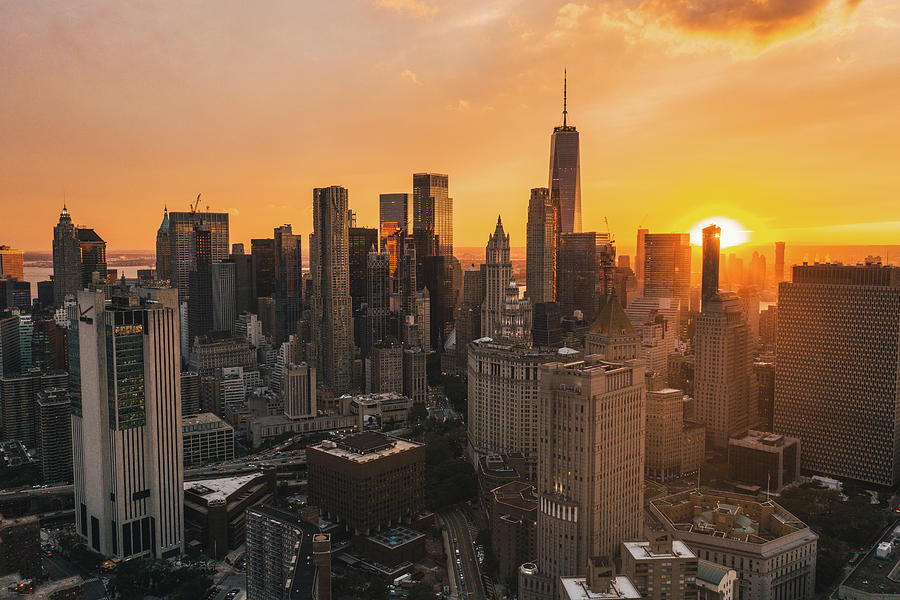The image showcases a vivid aerial view of a bustling city during sunset. Dominated by multiple tall skyscrapers, the scene is illuminated with an intense orange hue, progressively blending into yellow on the horizon, while a hint of blue is visible at the top left of the sky. The setting sun, about halfway below the horizon on the right side, casts a rich glow that contrasts with a dark cloud positioned on the upper right. Among the array of buildings, the tallest skyscraper stands prominently in the center background, distinguishable by a long spiky structure or possibly a tall pole atop it. Additionally, on the right side, there's a notable large building with a distinct checkered design. In the lower portion of the image, a highway with several cars is visible, further emphasizing the city's dynamic essence.